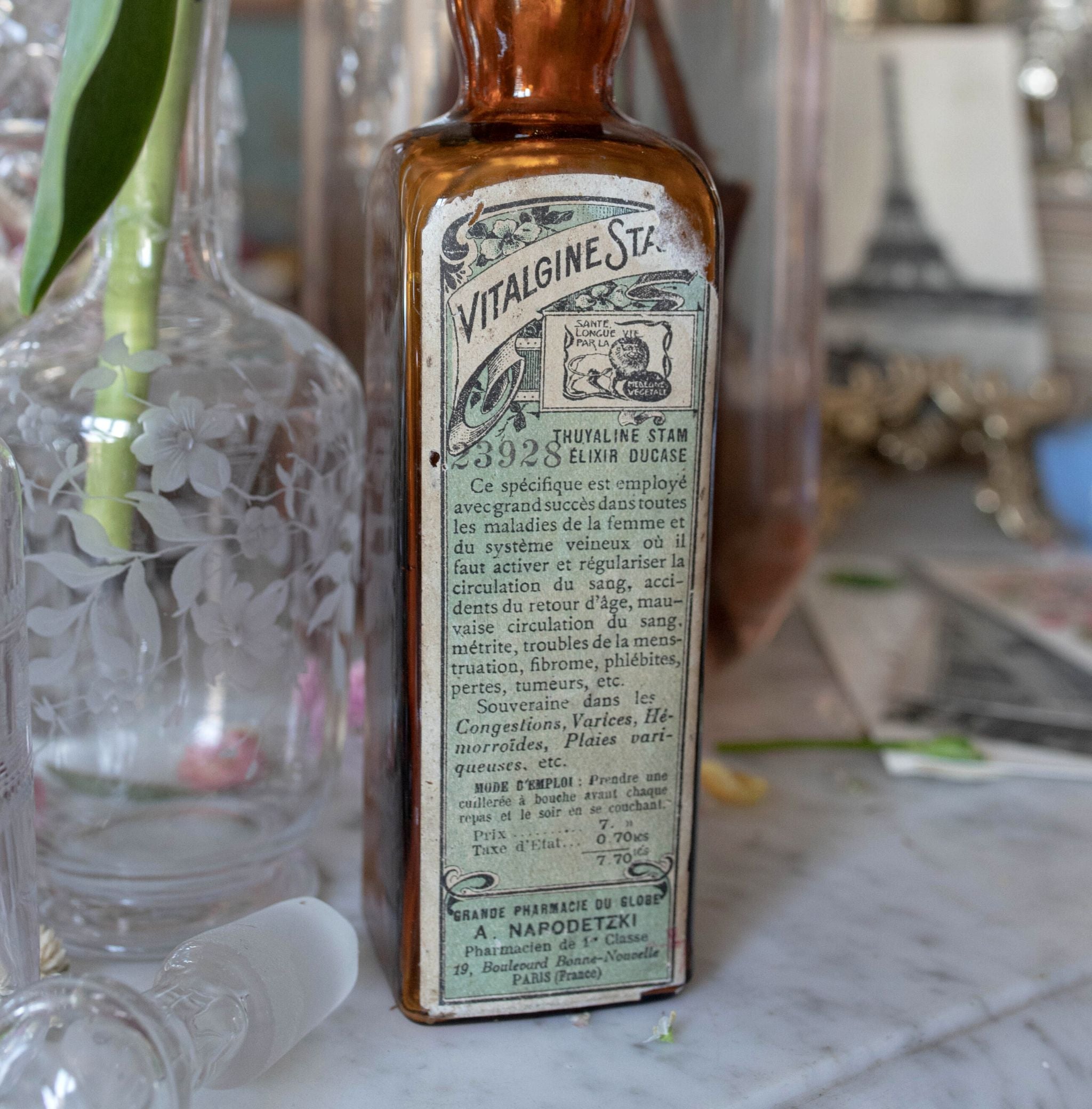The detailed image depicts a scene set on a white and gray marble countertop. Positioned to the left is a clear glass vase with an engraved floral pattern in white and gray frosted designs, showcasing a lone green plant stem extending from it. In front of the vase lies a glass bottle stopper. To the right is a vintage-style, amber-colored liquor bottle with a rectangular base that curves into a rounded top, partially cropped out of the frame. This bottle features a torn light green label bordered in white, with the legible text "VITALGENE STA" at the top, followed by a paragraph of foreign language text. Despite the label's damage, additional fragmented words remain visible, including "THOLULANE," "STAM," "ELIXIR," and "DUCASE."